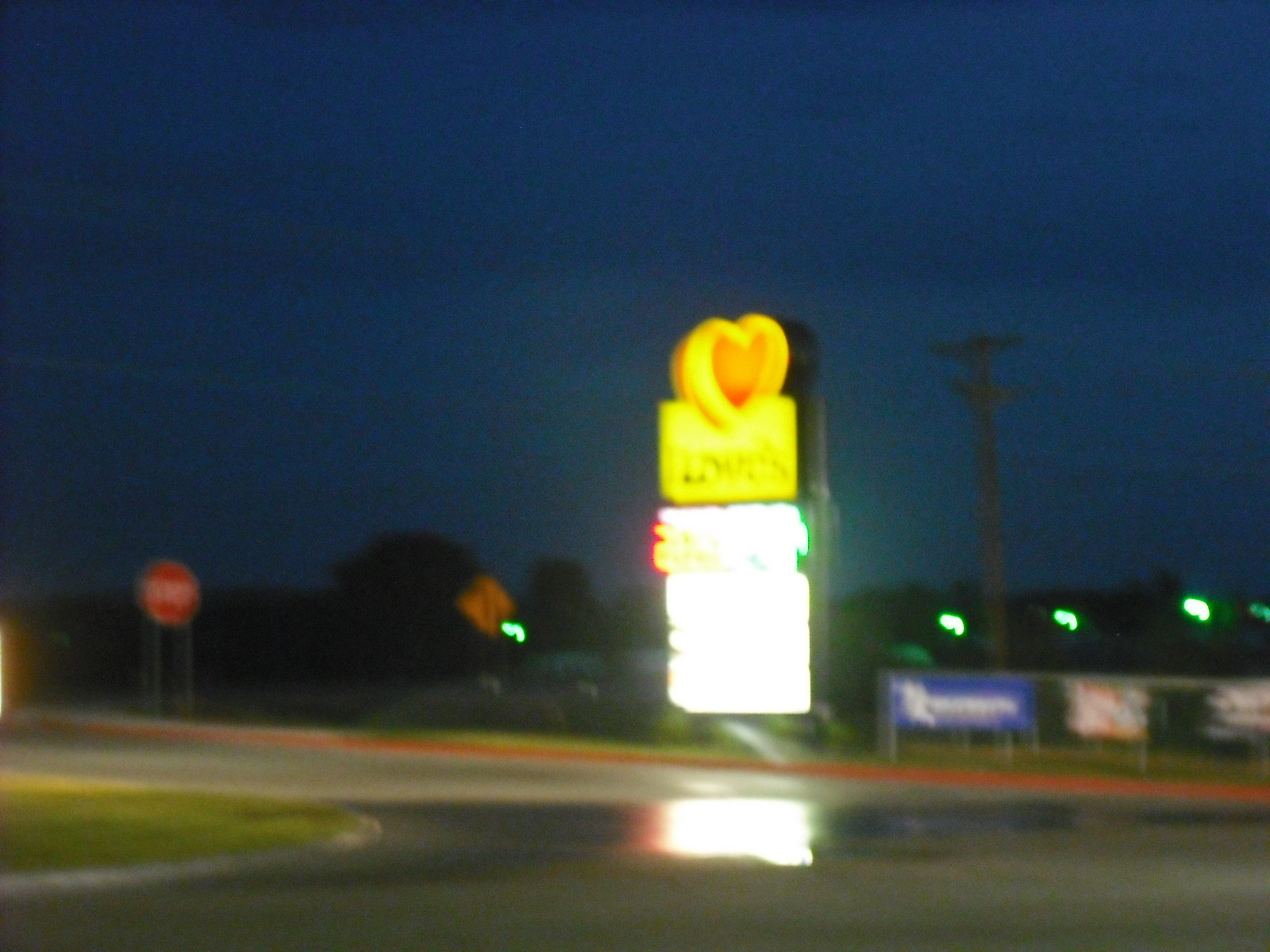In this blurry night-time photograph, the scene is captured from either a road or a parking lot, positioned across from the central focus of the image. The night sky forms a deep blue backdrop that contrasts sharply with the illuminated elements in the foreground. The road depicted makes a turn and is visibly flooded with water, creating a reflective surface.

Prominently featured across the street is a towering neon sign that ascends several feet into the air. The lower portion of the sign consists of a bright white rectangle, likely displaying gas prices, with a discernible neon number "2." Above this, a yellow rectangle showcases a red heart outlined in yellow, accompanied by black letters that are unreadable due to the image's blur. 

In the background, a low, single-story building adorned with various neon lights crowns the scene, adding a glow that punctuates the night. Further up the road, a stop sign is faintly visible, marking the scene's end.